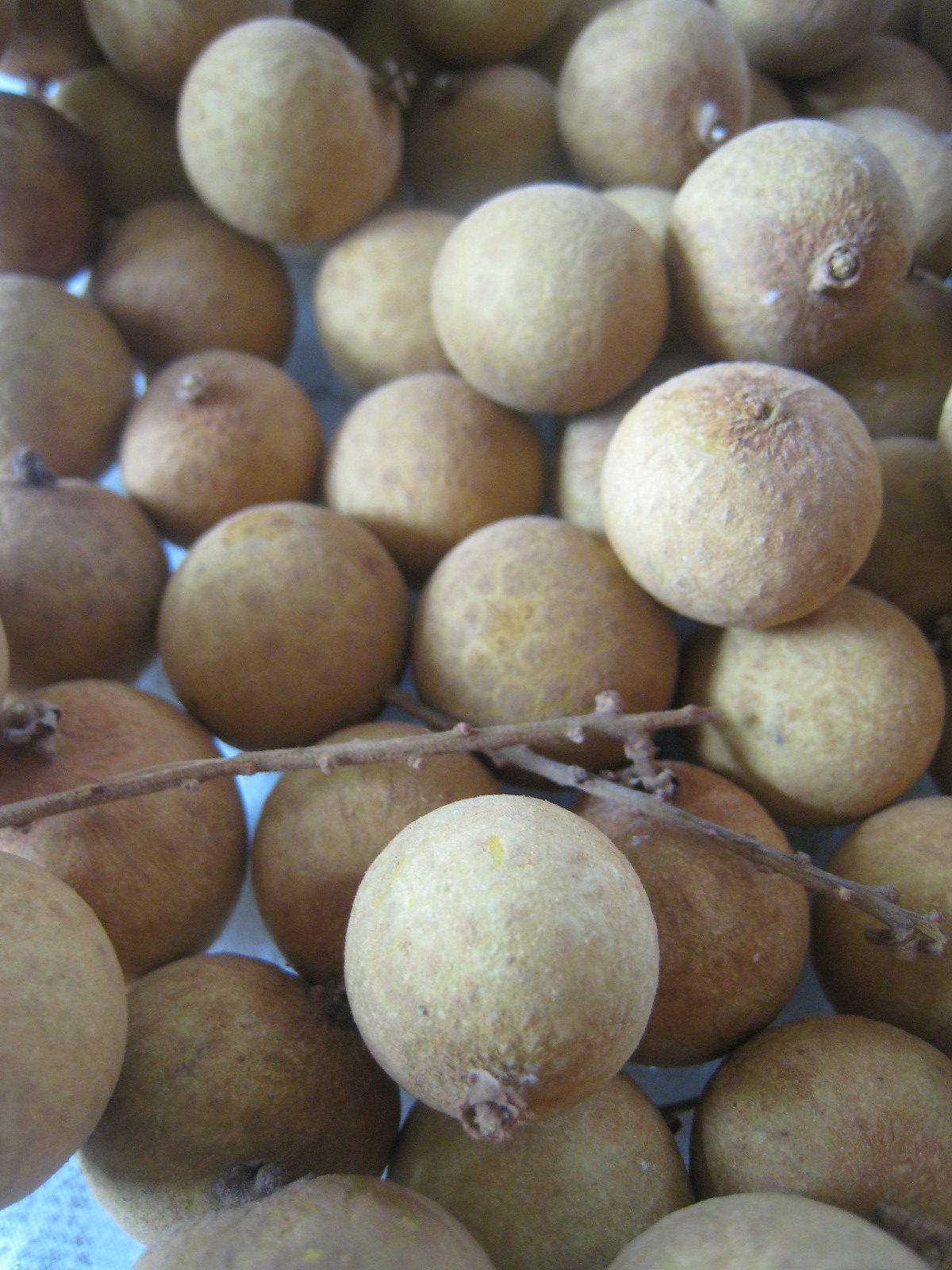This is an indoor photo displaying approximately 30 Logan fruits, also known as longans, scattered across a whitish-blue tabletop. The fruits have smooth, firm skins ranging from a pale camel color to various shades of cream and onion skin brown, some with speckled patterns. Two small branches are visible: one extending from the left and another from below towards the right, positioned slightly below the center of the image. Each fruit features a distinctive dimple on one end, indicating where they were once attached to their tree.